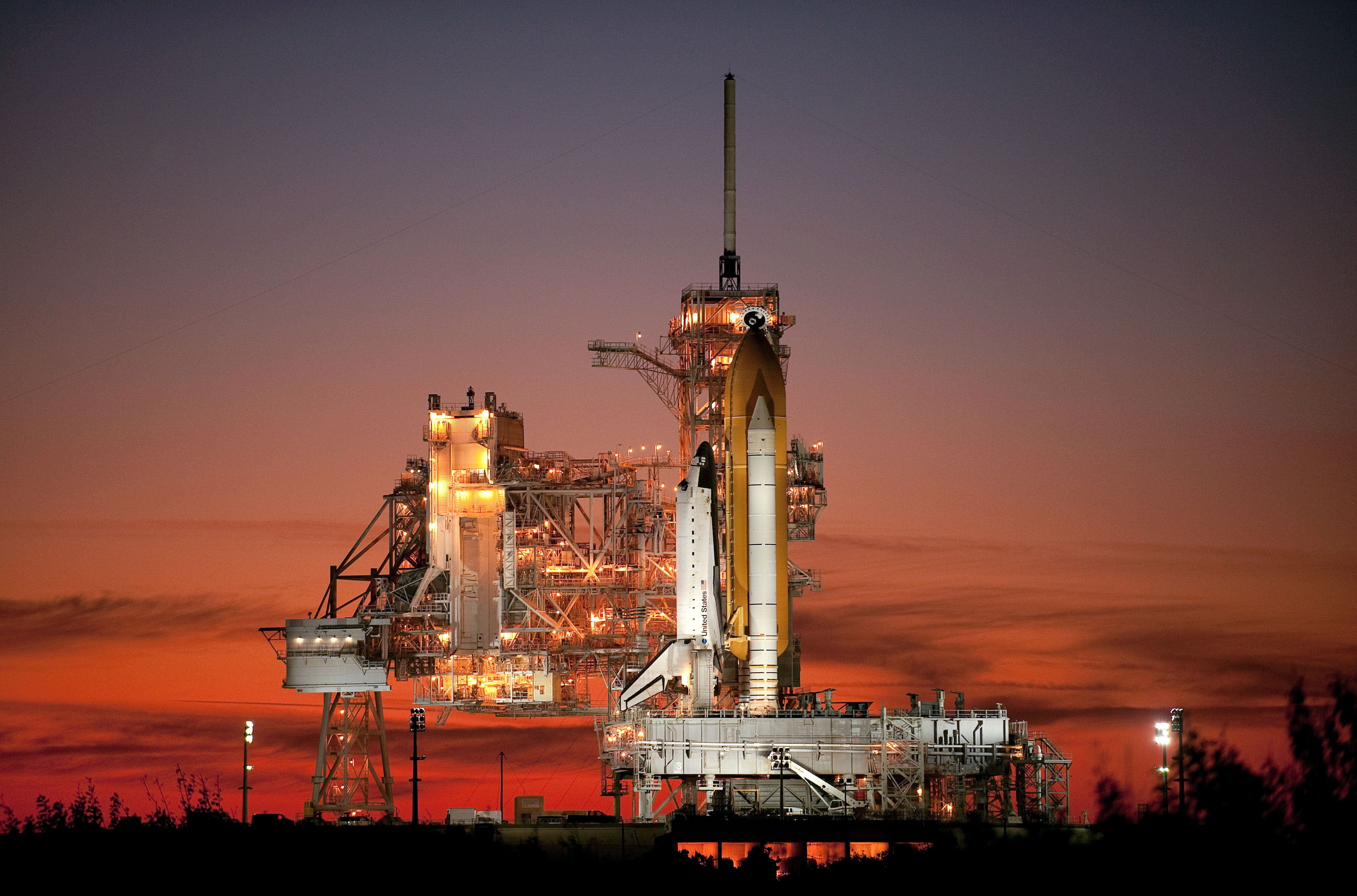In this detailed image, we observe the space shuttle poised on its launch pad, taken during the evening as the sun is nearly set, casting a breathtaking array of colors in the sky. The upper portion of the sky transitions from deep orange and yellow hues to a dark blue as night approaches. The large, rectangular launch pad is distinctly silver, held up by substantial steel legs and surrounded by intricate steel scaffolding.

At the center of the launch pad, there's a prominent burnt orange rocket, featuring an imposing white rocket thruster on its side with a sharp, pointy nose cone. Attached to this rocket, on the left side, is the majestic space shuttle, predominantly white with notable black details – a black strip on the top of the tail wing and a black nose cone. The space shuttle proudly displays the words "United States" along its body accompanied by a depiction of the American flag.

In the background stands a towering control structure, essential for the rocket's preparation and movement. This towering construction brims with numerous metal floors and levels, interconnected with steel girder support beams, giving it a complex, industrial appearance.

Overall, this image is rich with elements, showcasing the intricate setup and powerful grandeur of a space shuttle ready for launch amidst a captivating skyscape.